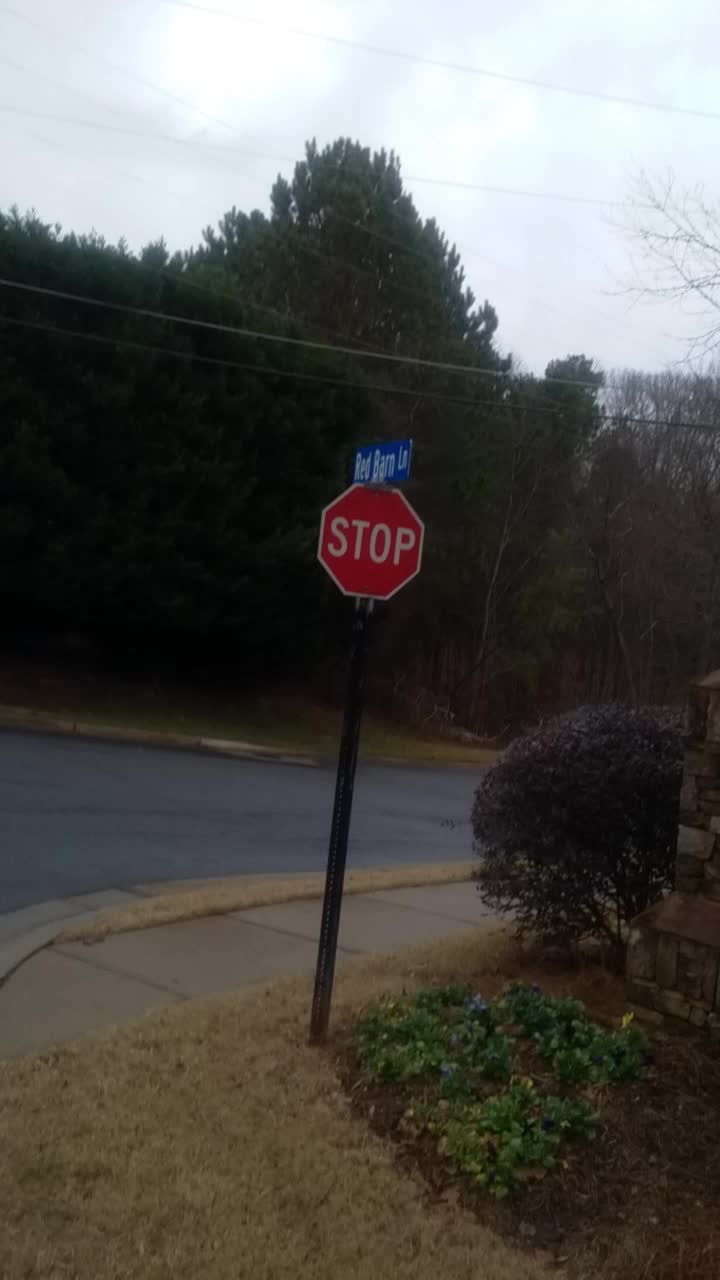This photograph captures a slightly skewed, angled view of a suburban American street in low lighting conditions, likely during the evening or underexposed. Central to the image is a standard red octagonal stop sign with white lettering that reads "STOP," mounted on a black pole set in a bed of dying golden grass. Above the stop sign is a blue street sign with white lettering that reads "Red Barn LN" for Lane, which is slightly turned to the left, making it difficult to read completely. To the right of the pole is a mulch bed lined with small, dark green plants, a black bush, and rocks. Adjacent to this is a larger bush, which appears dark, almost purple in the dim light. The foreground features a gray sidewalk beside a street curb with patches of yellow paint, leading into a roadway. Across the street, a line of dark green conifer trees can be seen, some still retaining leaves while others are bare due to the season's change. The background highlights a partly cloudy blue sky with some white clouds and the tops of trees, suggesting a mix of evergreen and deciduous varieties.